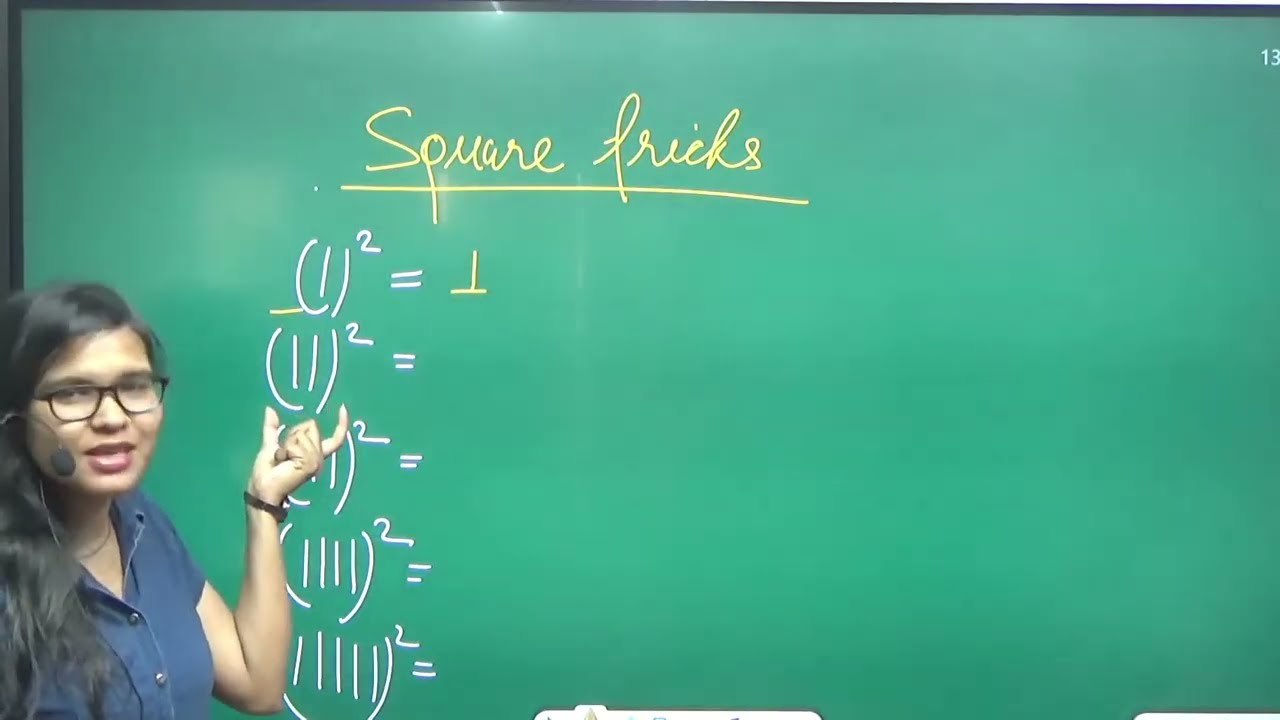In the image, a young woman of Indian descent stands towards the lower left corner in front of a large green chalkboard. She has dark brunette hair, parted on the side, and wears black horn-rimmed glasses. Dressed in a short-sleeved blue button-up shirt, she is equipped with a thin headpiece microphone, which is positioned near her mouth. She is gesturing towards the chalkboard with her left hand, while her right hand rests below a partially completed equation: "2 squared" written in parentheses. Notably, there is handwritten text in gold or yellow chalk at the top of the board that reads "Square Tricks," with an underline. Below this header, there are a few equations written in white chalk in a vertical sequence, starting with "1 squared equals 1," followed by "2 squared," "3 squared," and other unfinished formulas. The rightmost two-thirds of the image remains void of any writing, adding to the focus on the woman and the handwritten chalkboard text. The scene captures a teaching moment, with the woman actively engaged in explaining mathematical concepts.